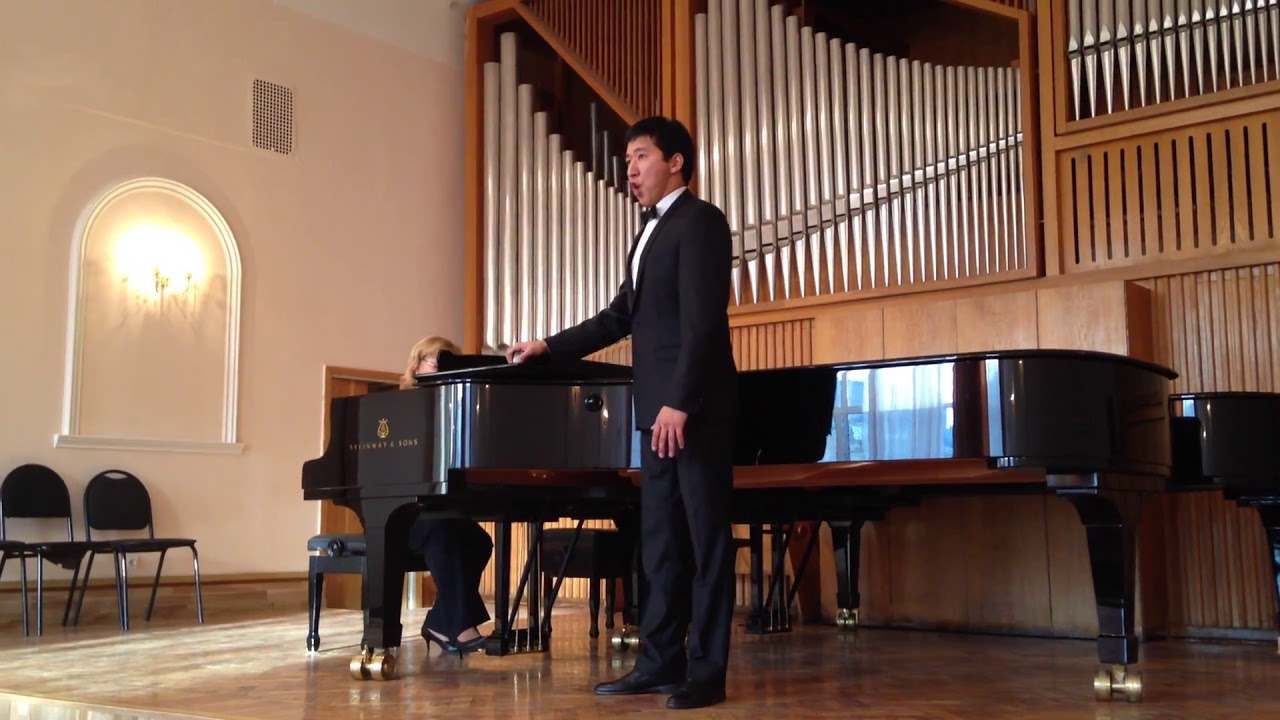This detailed image captures a poised music recital in an indoor concert hall or music room. Central to the composition is a large black grand piano adorned with gold printing, viewed from the back and side. A young blonde woman, dressed in black with heels, is seated at the piano, though her face remains unseen. In the foreground, an Asian man dressed formally in a suit or tuxedo and a white shirt stands next to the piano, possibly singing. His right hand rests on the piano as he maintains an operatic posture.

The backdrop features an elaborate assembly of organ pipes stretching across the wooden wall, creating a grand setting. To the left, a green wall with an arched, ornate window and mounted candelabra lights adds a touch of elegance. Positioned beneath this window, two black chairs underscore the room's grandeur. The wooden floor adds warmth to the image, reflecting the natural light that suggests a daytime performance. The overall color palette consists of browns, blacks, yellows, and whites, contributing to the formal and sophisticated atmosphere of the performance setting.